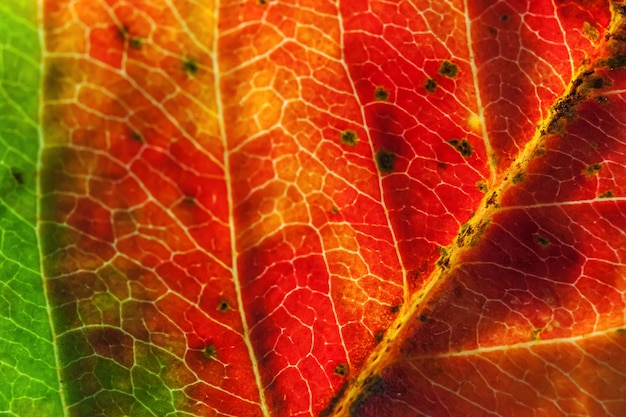This incredibly detailed, macro close-up photograph showcases the underside of an autumn leaf, with a focus on its vibrant and dynamic color palette. Starting from the left, the leaf exhibits a bright green hue that transitions into captivating shades of red, orange, and yellow as it progresses towards the right side of the frame. The intricate network of veins is prominently displayed, revealing the leaf's internal structure with precision. The broader base of the leaf sits at the bottom left, and the tip extends beyond the top right corner. Strewn across the leaf, particularly along the central vein, are numerous small black spots. These could potentially indicate insects sucking the sap, age-related decay, or disease. The image is exceptionally textured, making the leaf's surface and its diverse vein patterns appear almost tangible. The photograph does not include the outer edges of the leaf, further emphasizing the detailed interplay of colors and textures within this section.